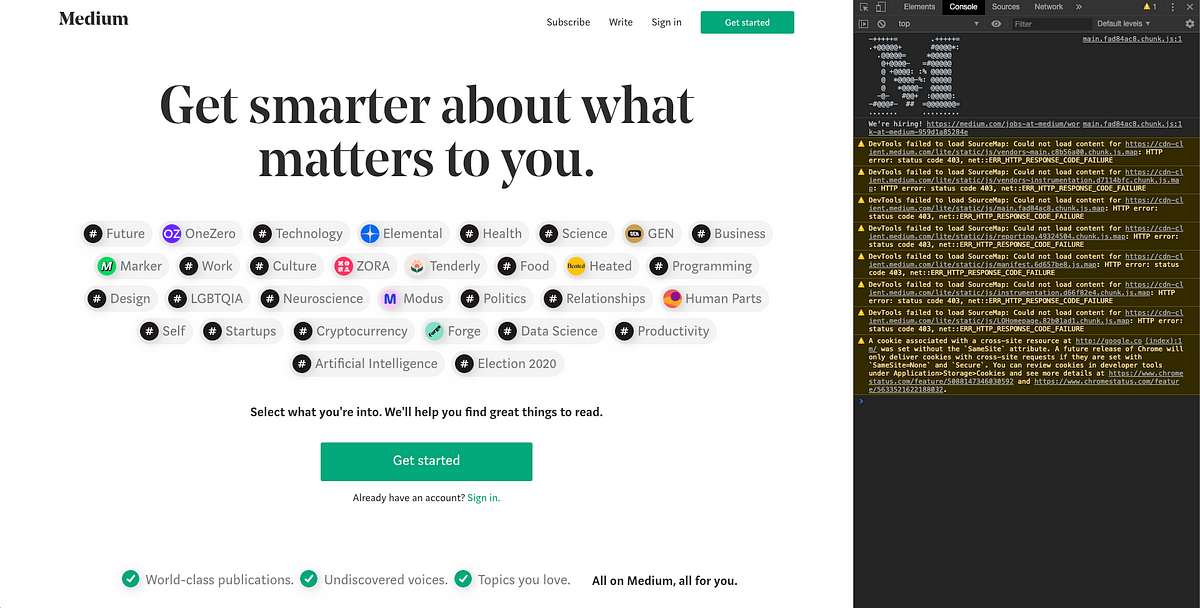This image depicts a white background, predominantly covering the right two-thirds of the screen. In the top left corner, the word "Medium" is prominently displayed. In the top right, navigation options are provided: "Subscribe," "Write," "Sign In," and a green "Get Started" button. 

The central portion of the image showcases the largest font, stating, "Get smarter about what matters to you." Below this, there's a section with various interest categories, each accompanied by a representative icon. The text instructs users to "Select what you're into. We'll help you find great things to read."

Following that, there is another green "Get Started" button. Underneath in smaller text, it prompts those who already have an account to "Sign In." The footer emphasizes, "World-class publications, undiscovered voices, topics you love, all on Medium, all for you."

Occupying the right one-third of the image, we can see what appears to be website code, likely from the element inspector tool, indicating the technical backend of the webpage. The small text makes specifics hard to read, focusing instead on displaying the technical intricacies.

Highlighted interest topics available for selection include:

- Future 1.0
- Technology
- Elemental
- Health
- Science
- Gen
- Business
- Marker
- Work
- Culture
- Zora
- Tenderly
- Food
- Heated
- Programming
- Design
- LGBTQIA
- Neuroscience
- Modus
- Politics
- Relationships
- Human Parts
- Self
- Startups
- Cryptocurrency
- Forge
- Data Science
- Productivity
- Artificial Intelligence
- Election 2020

Each topic is paired with an icon to facilitate easy selection for users to customize their reading preferences.